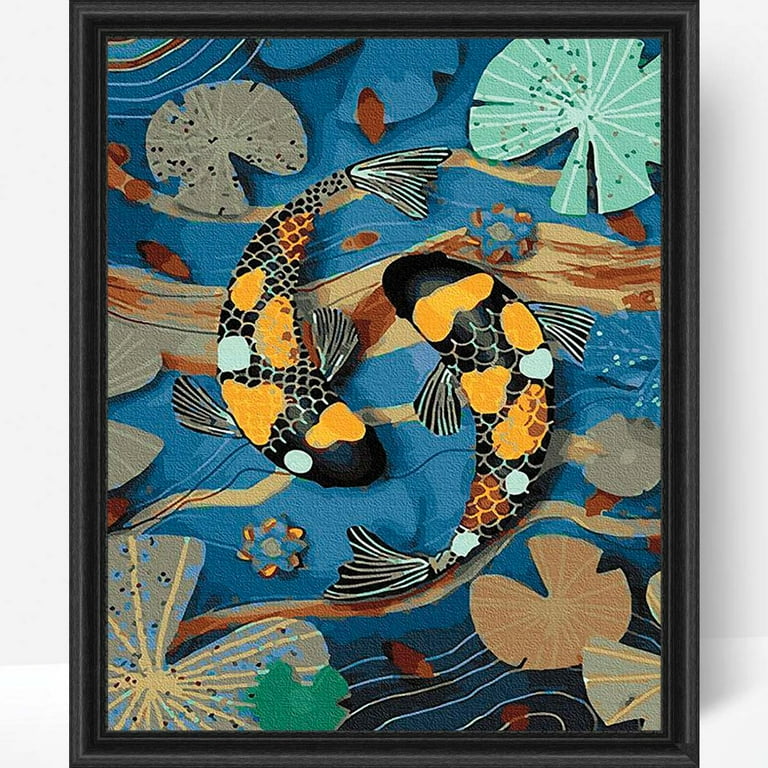This photograph showcases a striking painting framed in black, prominently displayed against a white wall. In the painting, two koi fish with black bodies adorned with orange, white, and yellow spots swim gracefully around each other in a dynamic circular motion reminiscent of a yin-yang symbol. The fish are captured with meticulous detail, including their white eyes, and are set in the center of the composition. The koi fish are surrounded by abstract, colorful swirls and waves that convey a sense of flowing water, including an extending wave pattern of orange and red that stretches horizontally across the painting. Additional elements like lily pads, illustrated with unique details such as yellow stripes and blue dots in the bottom left corner, add to the vibrant aquatic scene. The background features muted hues of blue and brown with various abstract shapes, possibly representing underwater plant life or other sea organisms, enhancing the overall artistic and animated feel of the painting.